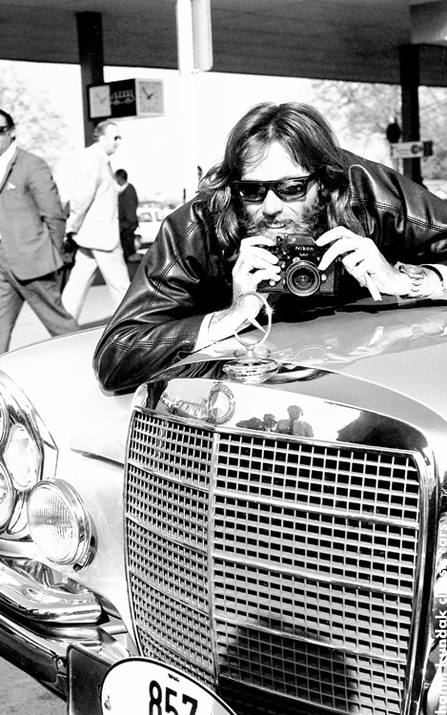In the black-and-white photograph, a man with long, flowy dark hair, a mustache, and a beard leans confidently on the hood of a car, which features a prominent large grill and the license plate bearing the number "857". He is dressed in a black leather jacket and sports dark sunglasses, enhancing his enigmatic aura. Clutched in his white hands is an old-school Nikon camera with a distinctive large circle in the center for focusing. A large watch also adorns his wrist. Behind him, three individuals dressed in suits are visible: one in a dark suit walking to the left, one in a white suit facing right, and another man in the distance looking away. The scene is set against a white background, adding a stark contrast to the central figure and the vehicle. There's a hint of a white car also visible in the background, emphasizing the monochromatic depth of the image.